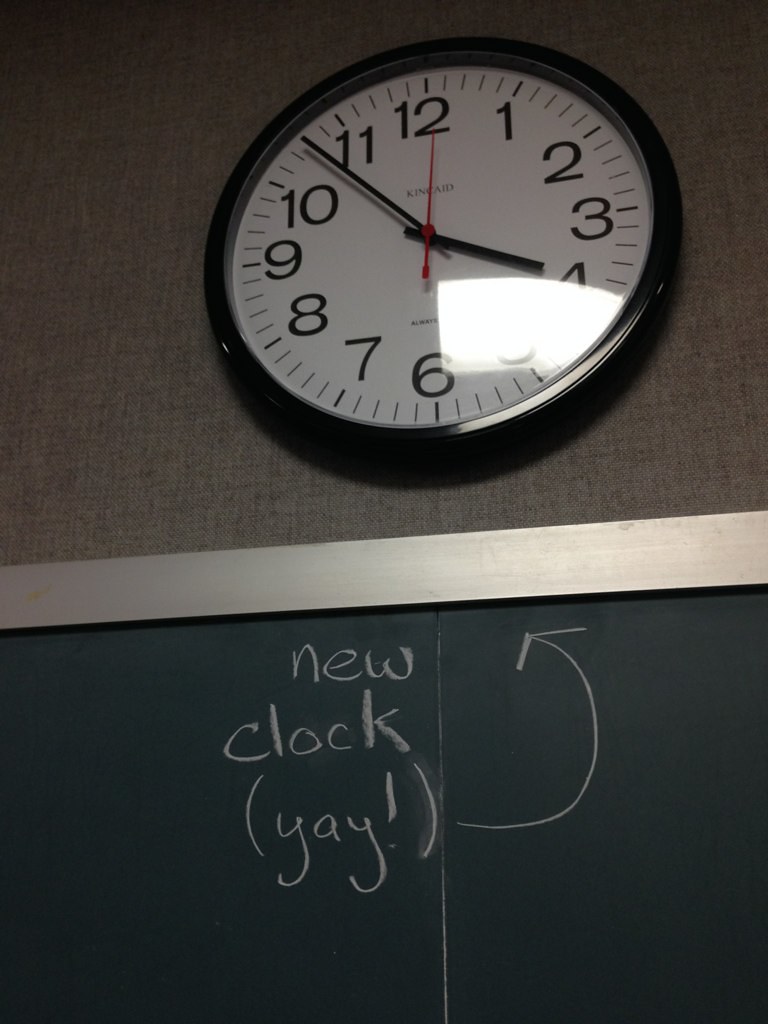This image features a large wall-mounted clock with a white face and black numbers. Each number is complemented by a line above it, with lighter lines indicating the minutes in between. The wall behind the clock appears to be made of a textured material resembling gray burlap. There is a noticeable reflection from a nearby window cast on the clock near the numbers 4 and 5. Below the clock, a bulletin board includes a blackboard with the handwritten message "New Clock (Yay!)" and a curly arrow pointing up towards the clock. A slim silver strip demarcates the space between the blackboard and the clock.